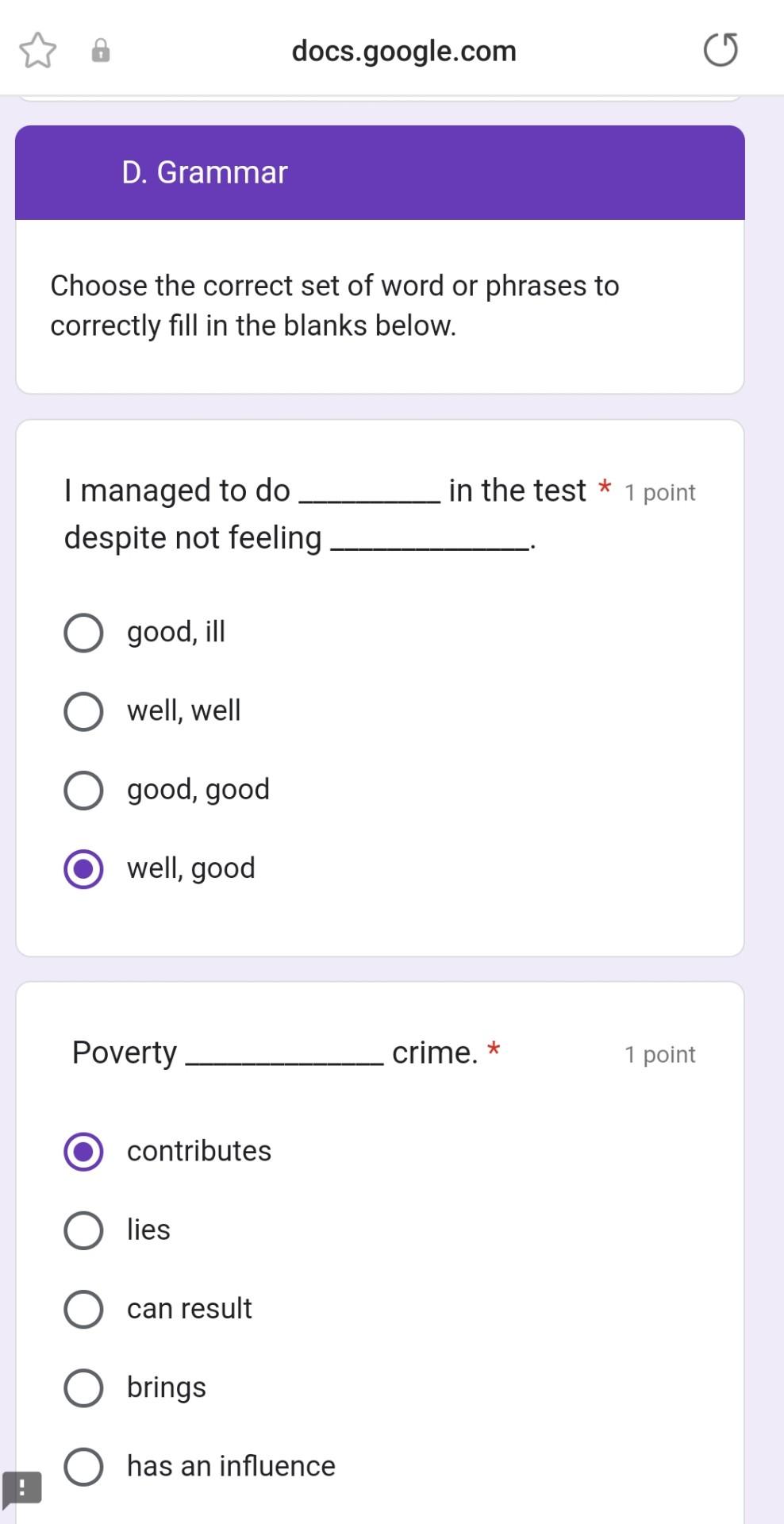This image captures a screenshot from a mobile phone displaying a section of a Google Docs document. The image orientation is vertical, being taller than it is wide, typical of a smartphone screenshot. The screen is slightly cropped at the bottom, omitting some minor details. 

At the top of the screen, there are several icons: a star, a lock icon, and a refresh symbol positioned in the upper-right corner. The URL `docs.google.com` is visible, indicating that the document is hosted on Google Docs. The interface includes a light lavender background with rounded white text boxes.

The uppermost white box features a dark purple banner with the text “D grammar” in white font, which appears to be a title or header. Inside the white area of the box, instructions read, "Choose the correct set of words or phrases to correctly fill in the blanks." This indicates the content comprises grammar test questions.

Below the instruction, the first question reads, "I managed to do blank in the test despite not feeling blank," with possible answer choices including "good," "ill," "well," and combinations thereof. The person taking the test has selected "well or good," which is noted as an acceptable answer.

The second question states, "Poverty blank crimes," with options such as "contributes," "lies," "can result," "brings," and "has an influence." The test-taker has chosen "contributes" as their answer, also deemed correct.

Each question seems to be worth one point, suggesting this could be part of a homework assignment or a standardized test preparation activity conducted via Google Docs on a mobile device.